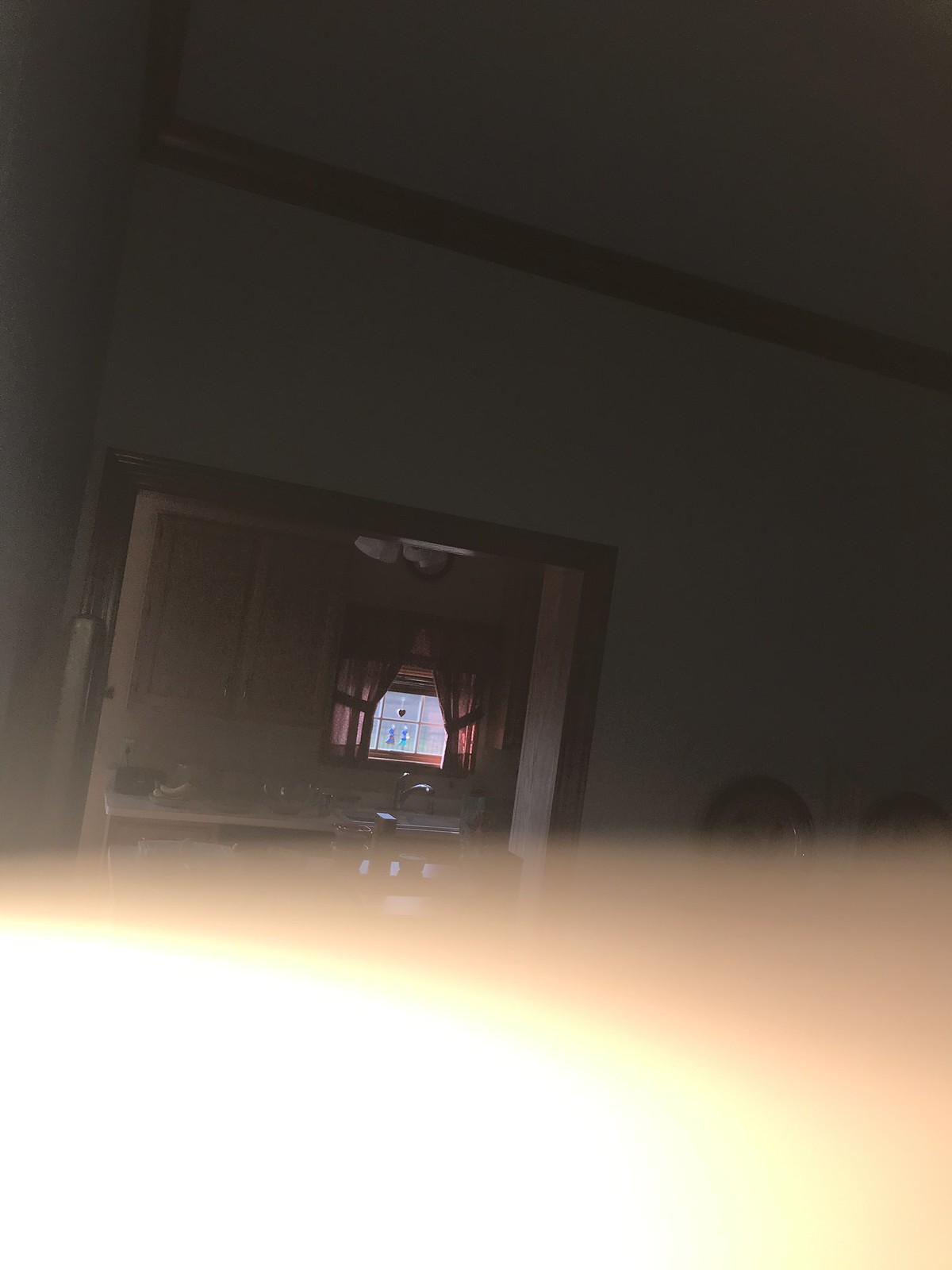The image, though somewhat poorly taken, captures the interior of a house. The bottom portion of the image is obscured by a solid white area blending into a peach-colored hue. Moving upwards, the scene transitions into what seems to be a living room. The ceiling and walls are white, accentuated by dark-colored trim and crown molding. There is trim around an open doorway that leads into another room. Through this doorway, a window is visible, featuring two characters with a red heart above them, dressed in purple and green. Below the window, a kitchen sink and part of a countertop are visible, suggesting this secondary room is likely a kitchen.